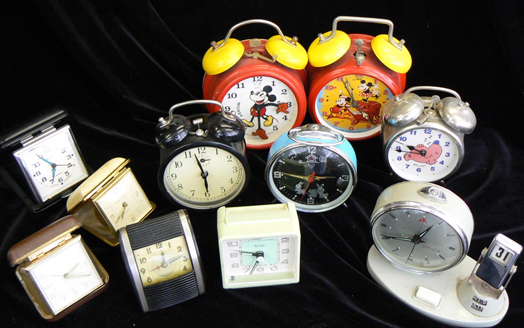This photograph showcases a diverse collection of vintage analog alarm clocks arranged on a luxuriant black velvet backdrop. Central to the display are various portable travel clocks, each distinct in color and design; a black one with a white face, followed by a smaller gold version, and another in dark brown with gold trim. A silver-framed clock with a yellowish center and black borders is situated nearby, alongside a pristine white square clock with black hands. 

Dominating the rear are classic twin-bell alarm clocks; a set of smaller black ones featuring white faces and silver handles, flanked by larger red counterparts with contrasting yellow bell components. Notably, one red clock incorporates Mickey Mouse, with his arms serving as clock hands, while the other features both Mickey and Minnie against a yellow background. 

Additional attention is drawn to a whimsical black and teal clock with a silver handle, another entirely silver with an indiscernible pink center detail, and a sleek, modern clock with a flat white face, black hands, and a refined silver trim on an oval platform, accompanied by a small silver rectangular box displaying the number 31 in black.

In summary, this intriguing assembly of timepieces ranges from quaint travel clocks to playful character-themed alarms, all steeped in nostalgia and meticulously detailed.